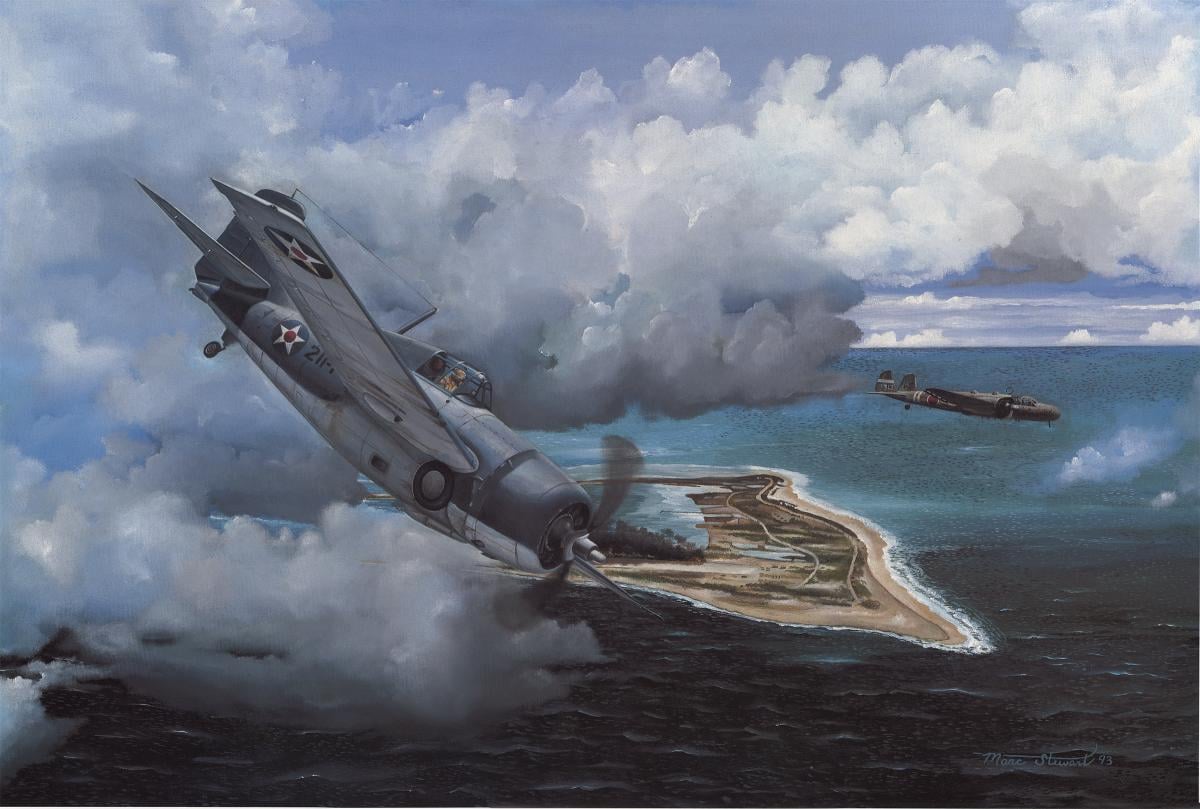This is a square watercolor painting set against a white background, featuring a serene scene of two military airplanes flying over calm, dark blue water. The sky above the water is filled with many white, fluffy clouds that envelop the planes. Near the center of the image, the closer airplane, which is blue and light gray in color, is facing downward and showcases a blue circle with a white five-pointed star and a red circle at its center on its side. In the background, we see the second airplane, smaller and farther away, depicted amidst the clouds or possibly smoke and exhaust trails. A small beige island can be discerned in the distance, adding a touch of terrestrial contrast to the composition. The detailed rendering of the aircraft and the tranquil water below provide a vivid juxtaposition, emphasizing both the isolation and the solidarity of the planes within the broad expanse of their surroundings.